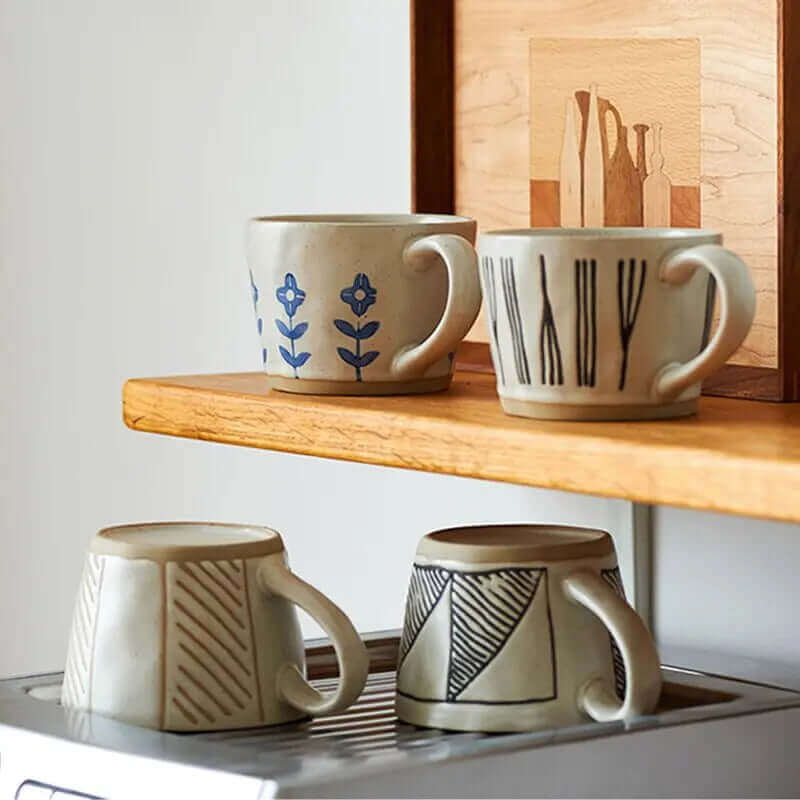This photograph showcases a display of four handcrafted ceramic teacups arranged on a wooden shelf and platform. The two teacups on the lower platform are positioned upside down. The teacup on the bottom left features a reddish-brown geometric pattern of stripes and lines on a white glazed background, accented by a beige rim. The bottom right cup displays an alternating pattern of black and white triangles, with the black triangles containing diagonal lines. Above these, on the wooden shelf extending from the right side of the image, are two right-side-up teacups. The upper left teacup is adorned with three evenly spaced blue flowers, each with four petals and two sets of four leaves connected by slim stalks. The top right cup showcases a repeating pattern of three-pronged forks and three vertical stripes, alternating in orientation around the cup. A wooden painting or carving of bottles is situated behind the upper shelf, adding an additional rustic element to the display. Each teacup, though white with distinct patterns, exhibits the charm of handmade ceramics, evident in their slightly uneven forms.